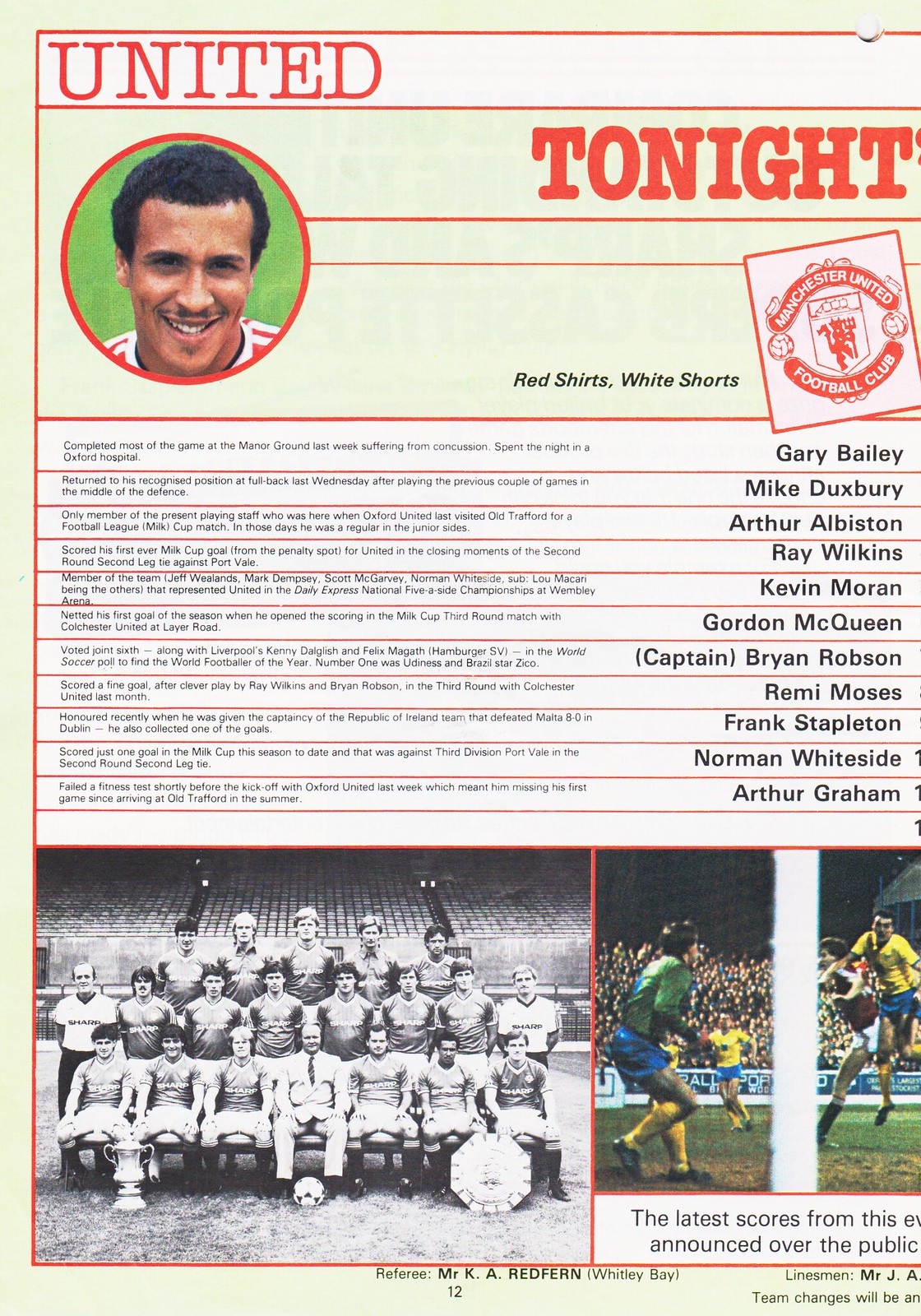A vibrant soccer poster, likely for a Manchester United match, greets us with bold red text reading "UNITED" at the top, followed by "TONIGHT" below it. A standout feature is a smiling soccer player with thick black hair, captured within a red circle to the left of the text, sporting a thin mustache and red stripes on his shirt.

Adjacent text reads "Red shirts, white shorts," tied together with the Manchester United Football Club logo. Below this, a meticulous list of team player names spans from Gary Bailey to Arthur Graham. 

Further down, vivid imagery unfolds with a black-and-white team photo on the left, portraying three orderly rows of players and staff seated in a stadium. On the right, contrastingly, a vibrant match scene captures one player in a yellow jersey seemingly about to score while a green-clad goalie leaps to block, set against a crowded stand.

A small white box at the bottom mentions the latest scores being announced over the PA system, though partially obscured. The overall background of the poster is light green, lending a cohesive and eye-catching design reminiscent of classic football heritage.